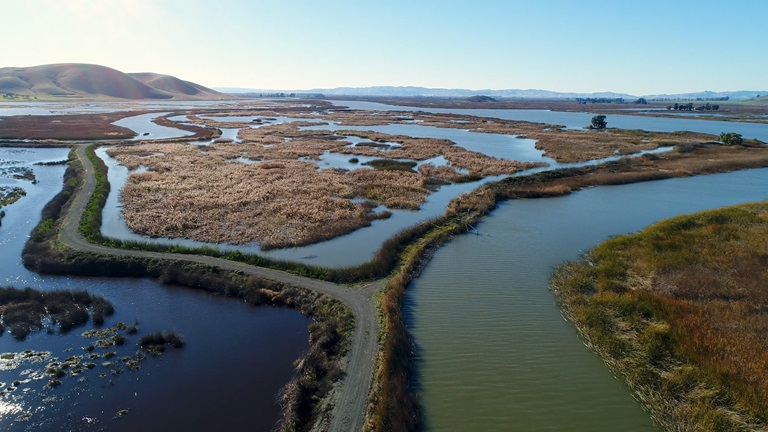An aerial view captures an extensive, natural wetland characterized by a mosaic of pools, varying shades of water, and patches of vegetation. A well-traveled, multi-lane gray asphalt road runs through the heart of the wetland on a small hill or dike, splitting off into a dirt side road that veers toward a grassy inlet. The left side of the image features the darkest pools of water, interspersed with clumps of vegetation, while sparse trees punctuate the yellowed and dark brown landscape. In the center, a little island with a few trees stands out amid the marshy expanse. The serene setting is topped off with a large, almost smooth-looking hill on the top left, under a light turquoise sky, adding to the natural, undisturbed beauty of the scene.